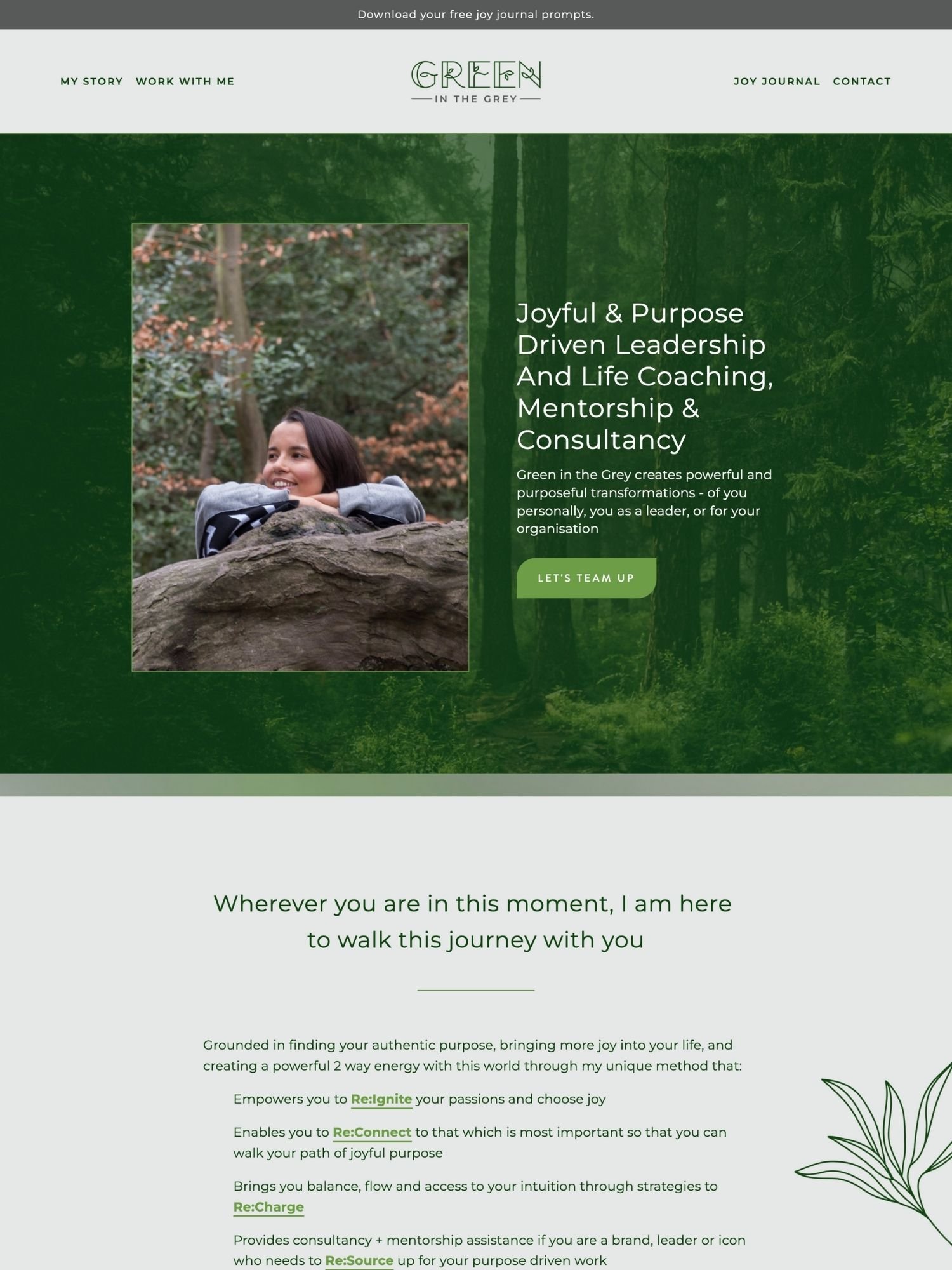The screenshot depicts a vertical webpage with a clean, user-friendly layout. At the very top, a thin, dark gray banner contains text that reads, "Download your free Joy Journal prompt." Below this banner, a light gray header bar features the logo "Green in the Gray," characterized by green trees and stylized text. To the left of the logo are navigation links labeled "My Story" and "Work with Me," while to the right are links titled "Joy Journal" and "Contact."

The main section of the page showcases a central translucent green screen superimposed on a forest background. To the left, there is a photograph of a smiling woman, her arms folded casually on a large rock. Adjacent to the image, bold text declares, "Joyful and Purpose-Driven Leadership and Life Coaching, Mentorship, and Consultancy." Beneath this slogan, a call-to-action button reads, "Let's team up."

The bottom portion of the page features a light gray background with green text and an illustration of a leaf in the lower right-hand corner. The heading reads, "Wherever you are in this moment, I am here to walk this journey with you. Grounded in finding your authentic purpose, bringing more joy into your life and creating a powerful two-way energy with this world through my unique method that..." Underneath the heading, explanatory text is provided along with four underlined green links for further navigation.